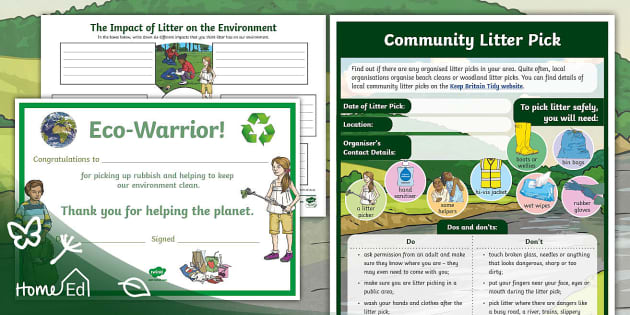This image presents an educational worksheet graphic titled "Community Litter Pick," designed to teach the do's and don'ts of picking up garbage. It's part of a teacher's packet published by Home Ed, indicated by their logo featuring silhouettes of a butterfly, a daffodil, and a leaf in a green triangle on the lower left corner. The worksheet includes designated spaces for filling out the date, location, and organizer's contact details for a litter pick event.

The graphic includes a section titled "The Impact of Litter on the Environment," illustrated with a cartoony picture of kids playing and picking up trash in a field. It serves as a visual aid to highlight the environmental impact of littering. Additionally, there is a list of essential items for a safe litter pick, such as litter pickers, hand sanitizer, high-vis jackets, garbage bags, wet wipes, and rubber gloves.

A printable award captioned "Eco Warrior Award" is also featured, with spaces to personalize it with a recipient's name. The award displays images of individuals picking up trash and carries a congratulatory message: "Congratulations to [blank] for picking up rubbish and helping to keep the environment clean." This comprehensive packet provides valuable tools and resources for teachers to educate students about environmental stewardship and community involvement in litter picking.